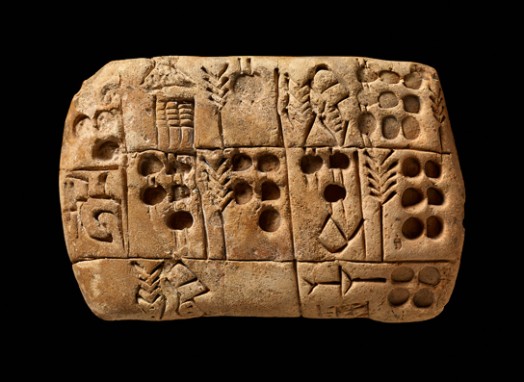The image features an ancient artifact reminiscent of archeological finds, set against a stark black background. This relic, possibly a rock tablet, has a rectangular shape with rounded edges and a chocolate brown hue. The surface is adorned with numerous carved symbols and patterns, resembling hieroglyphics, which suggest it could have been used as a communicative tool in ancient times. There are various round holes scattered across the tablet, particularly in the center, top right quadrant, and bottom right quadrant. These holes and the intricate designs create a grid-like structure, separating different sections of the tablet. The detailed carvings and weathered appearance of the tablet emphasize its historical significance.